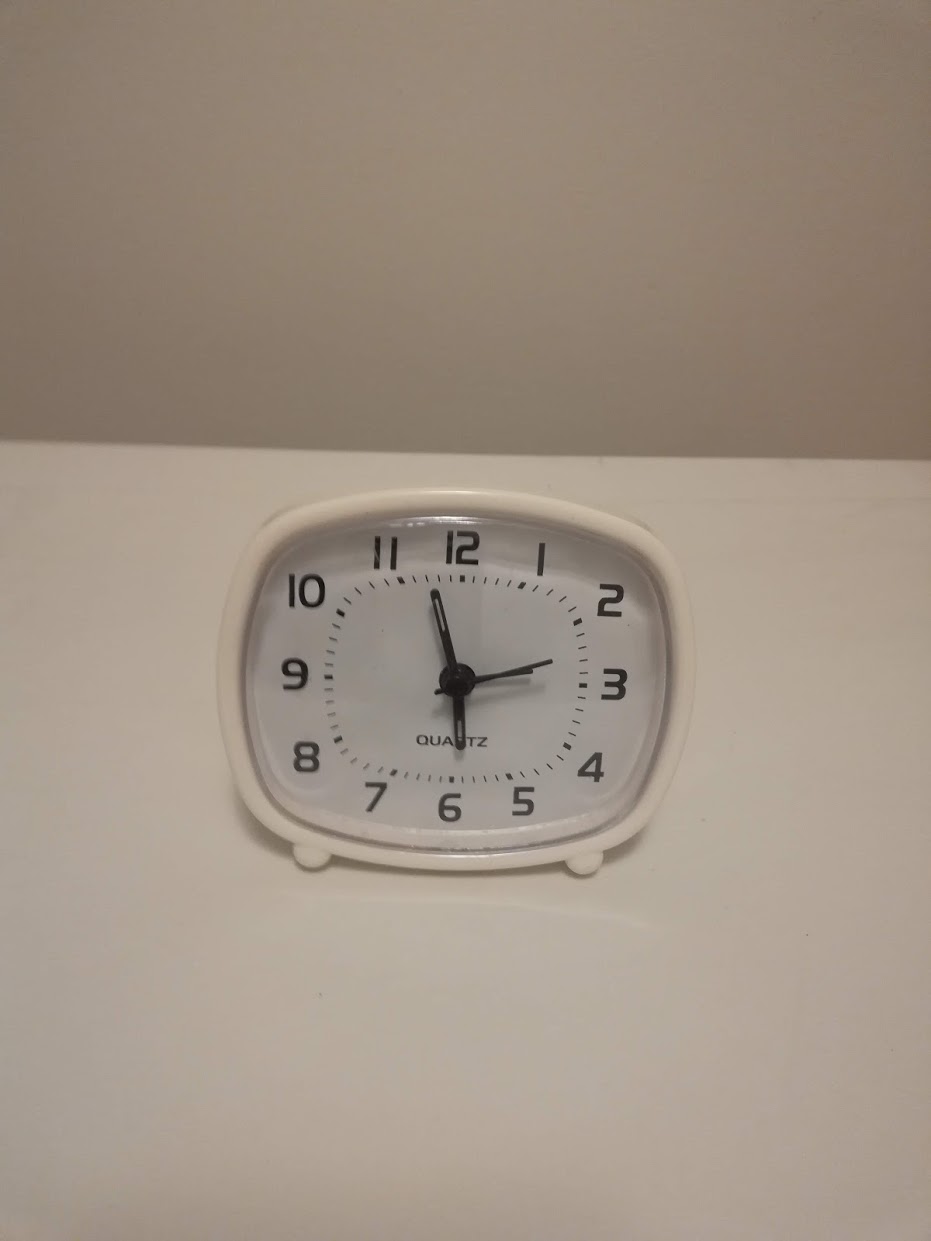The image features a small, white plastic-cased clock that is likely positioned on a table, given the presence of two round plastic feet visible between the numbers four and five, as well as seven and eight. The clock displays a time of approximately 5:57, with the second hand positioned between the two and three. The background consists of a darker gray, contrasting with the off-white surface on which the clock rests, suggesting a minimalist and modern setting. The angle of the photo introduces some ambiguity, hinting that the clock could either be viewed slightly from below or at eye level, adding an intriguing element to the composition.